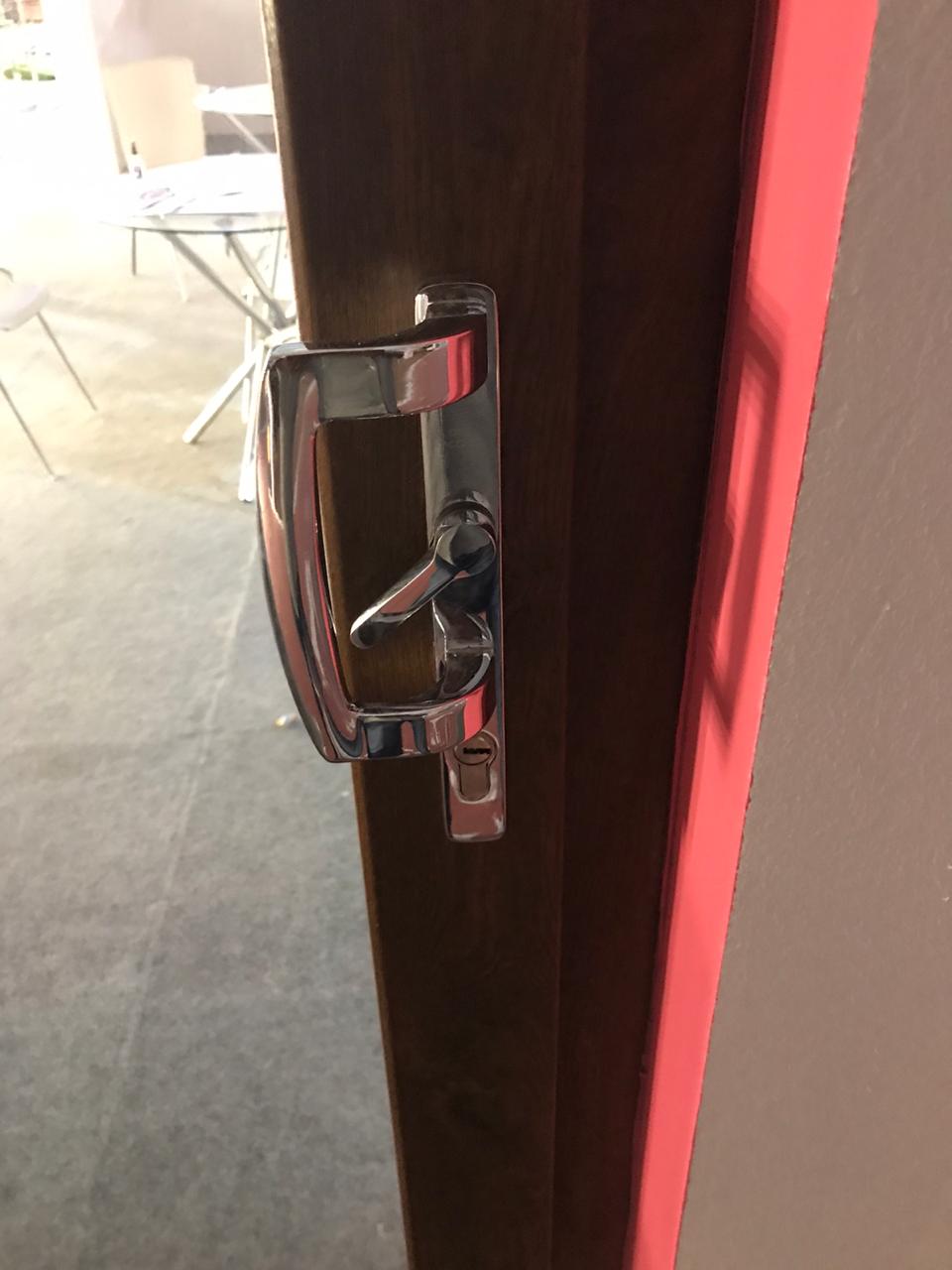This is a close-up, color photograph of a heavy-duty, chrome door handle on a sliding glass door. The handle is metallic and features a central lever for locking the door. The frame around the glass panel is made of dark mahogany wood. To the right of the door, the wall is trimmed in white with a visible red section. Through the glass door on the left side of the image, there's a view of an outdoor area that includes a white walkway, a round glass-top table, and white chairs, likely set on a gray stone patio or an outside slab. This setup suggests that the door leads to a shaded outdoor space.